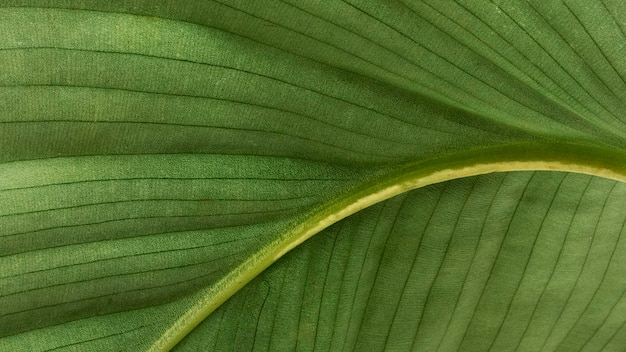This image is a highly detailed close-up of a green leaf, prominently featuring intricate vein patterns. The leaf, illuminated by what appears to be yellow sunlight from underneath, spans the entire frame, showcasing its vibrant green hues. The main stem runs diagonally from the right of the image to the lower left, segmenting the leaf into sections with veins running both horizontally and vertically. The interplay of lighter and darker greens highlights the thick, elongated sections of the leaf, underscoring its lush and robust nature. Overall, the leaf is the sole focus of the image, dominating the scene with its detailed texture and vivid color.